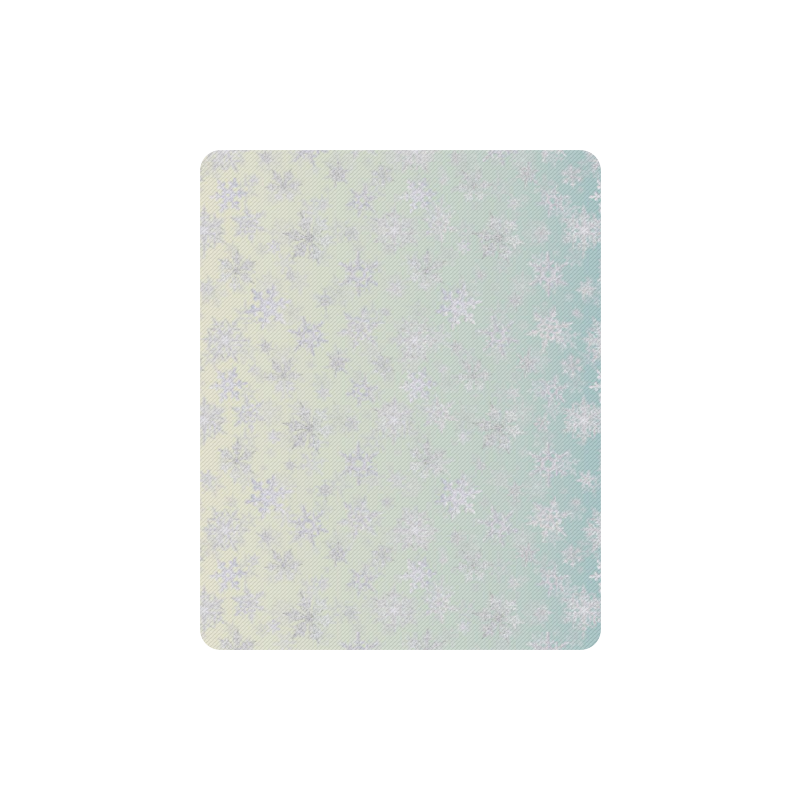In this detailed description of the image, the central focus is a piece of material, possibly wallpaper or a bathroom mat, featuring an intricate, winter-themed design. The material has a background that transitions from a light greenish-blue on the left to a deeper, more saturated aqua on the right. The surface of the material is shiny and iridescent, which gives it a shimmering, metallic appearance. Scattered across this background are finely detailed white and silver snowflakes, each unique in design with varying shapes and sizes, ranging from star-like forms to those resembling real snowflakes. The overall arrangement of the snowflakes is random, adding to the non-repetitive feel of the pattern. This image is portrayed in a color photograph with portrait orientation, showcasing the subject—a rectangular piece of shiny, decorative material with rounded corners—centered against a neutral backdrop. The style conveys a winter mood, with the radiant blend of colors and reflective qualities enhancing the intricate snowflake designs.